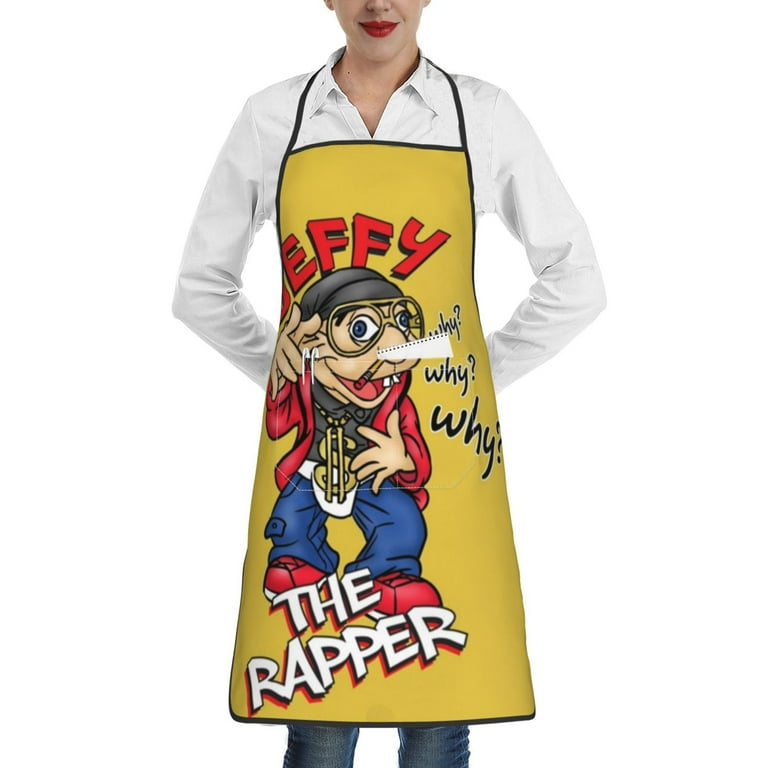A professionally-taken photograph depicts a woman, likely in her 20s or 30s, set against a stark white background that suggests a studio setting. The image is cropped from the bridge of her nose to her knees. She has red lipstick and fair skin and is wearing a white open-collared shirt with her hands placed behind her back, elbows bent outward. She is also wearing blue jeans. The woman dons a distinctive yellow apron with black outlines around her neck. The apron features a whimsical cartoon figure of a rapper. The figure sports exaggerated glasses resembling goggles, a dark gray shirt, blue jeans, and red shoes. His mouth is wide open, revealing two prominent buck teeth, and his hands are raised with fingers splayed as if making hand signs. He wears a gold dollar sign necklace around his neck. Above the cartoon character, large letters spell out "EFFY," although the first letter is partly obscured by the apron wrapping around her waist. To the right side of the apron, vertically aligned, are three instances of the word "Y" in dark blue, each followed by a question mark. Diagonally across the bottom of the apron in white letters is the phrase "The Wrapper," completing the playful and detailed design.